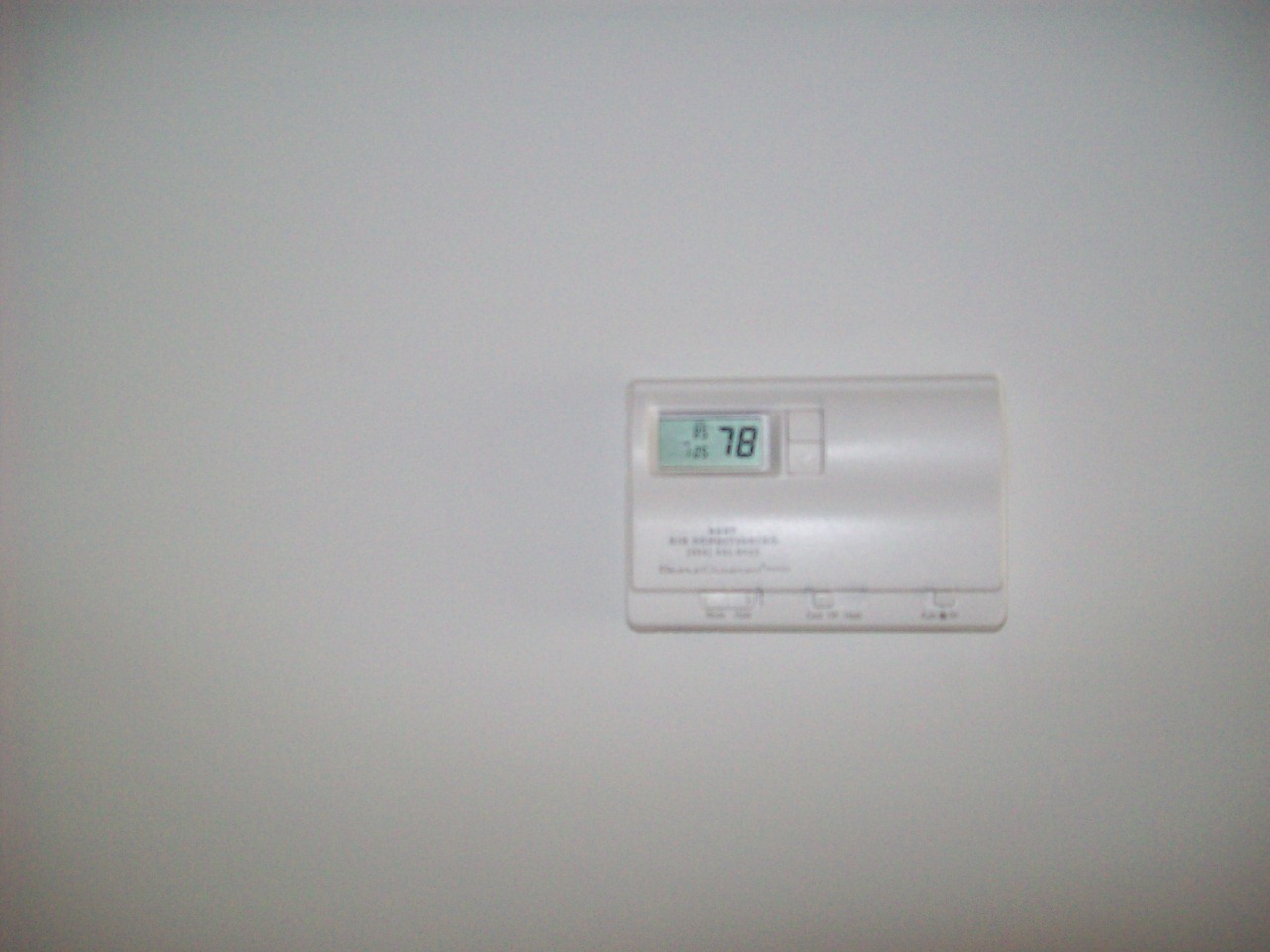A photograph captures a white thermostat centrally mounted on a wall, which, due to the shadowing in the image, appears almost gray. The thermostat is rectangular and features a small rectangular display in the upper left-hand corner, showcasing the temperature "78" in black on a light gray background. To the right of the display is a button that seems to be toggled upwards. The bottom left corner of the thermostat has four lines of illegible, blurry writing. Below these, a lower band is divided into three sections, each containing toggle buttons. One section likely serves as an on-off switch, while the other two have options that are too small and blurry to decipher.